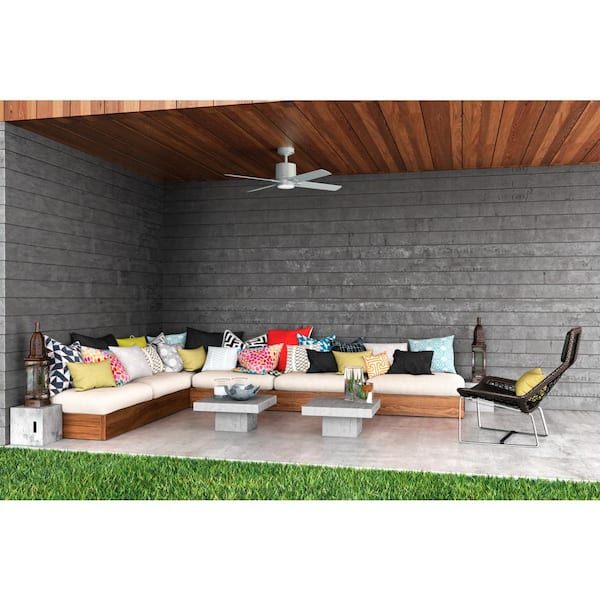This horizontal color photograph captures a well-maintained backyard that features a lush expanse of grass in the foreground. The central focus is a recessed patio area extending from the house. The patio is defined by gray brick walls and a marble floor, creating a sophisticated backdrop. Alongside the gray brick wall runs a spacious, L-shaped sectional couch. This couch is adorned with an array of approximately 20 pillows in a lively mix of black, red, white, and light blue hues. The couch comprises two sections: the left side has two white cushions, while the other section has three, all seamlessly integrating into the L-shape.

In front of the couch are two low, gray, marbled coffee tables that add to the modern aesthetic of the space. Additionally, there is another chair positioned to face the sectional, distinguished by a bright yellow pillow. The cozy yet elegant setup features a couple of decorative lanterns, enhancing the lounge ambiance. All of this is sheltered under a brown, wooden roof, from which a white ceiling fan hangs, providing a breezy atmosphere perfect for relaxation.